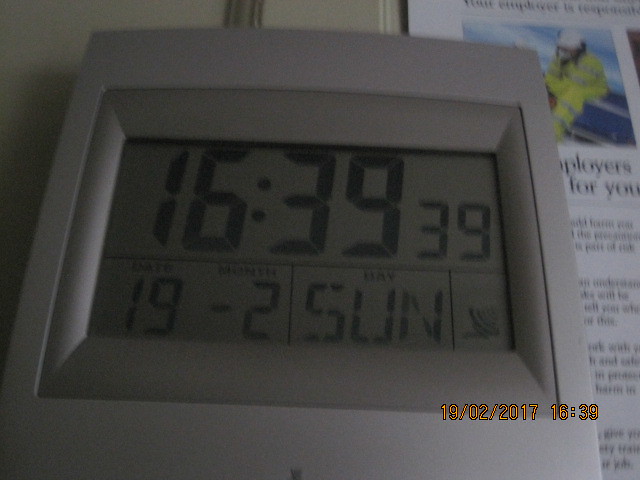The image is a close-up photograph of a digital alarm clock. The outer borders of the clock are white, while the inner frame is silver. The display shows black digital numbers against a greenish-gray background. The main time displayed is "16:39:39", indicating the time in hours, minutes, and seconds. 

Below the time, there are three distinct sections separated by black lines. The leftmost section displays "19-2" with labels above the digits indicating "DATE" for 19 and "MONTH" for 2. To the right, the next section shows "SUN," abbreviating Sunday, with "DATE" labeled above it. The final section contains an unidentifiable symbol not fully visible in the image.

At the very bottom of the display, additional text reads "19-02-2017 16:39", indicating the full date and time once more: 19th of February, 2017 at 16:39.